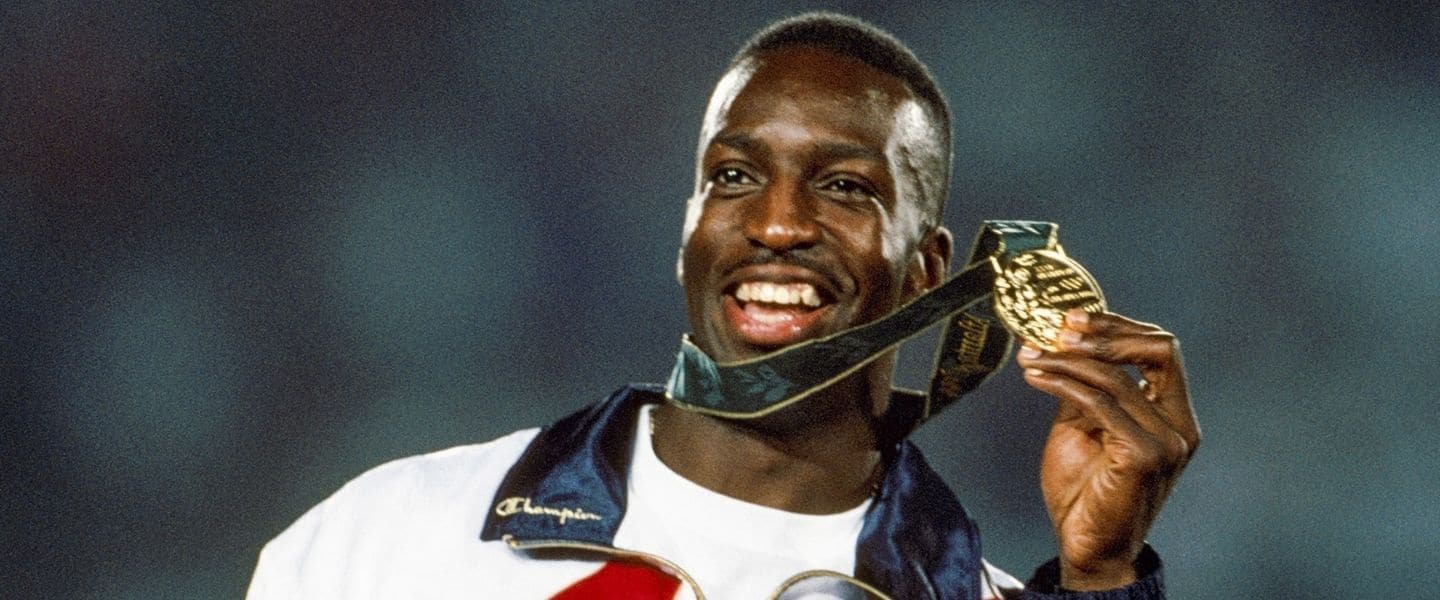This is a close-up, full-color photographic image of a jubilant black man taken outdoors, likely at night. He is smiling broadly, showcasing a lot of white teeth, and directs an enthusiastic gaze at the camera. The man holds up a gold medal with his left hand, positioned at face level, the medal hanging from a black strap around his neck. His attire consists of a white Champion brand jacket adorned with red markings and a blue or black collar, featuring the word "Champion" and the Champion logo emblazoned on the left side. His skin glistens under the lighting, particularly around his temples, suggesting the presence of a flash. He sports a closely-cropped haircut and a high forehead. The background is a blurred mix of gray with black splotches, keeping the focus on the man and his triumphant expression. The image is horizontally rectangular and lacks a border.